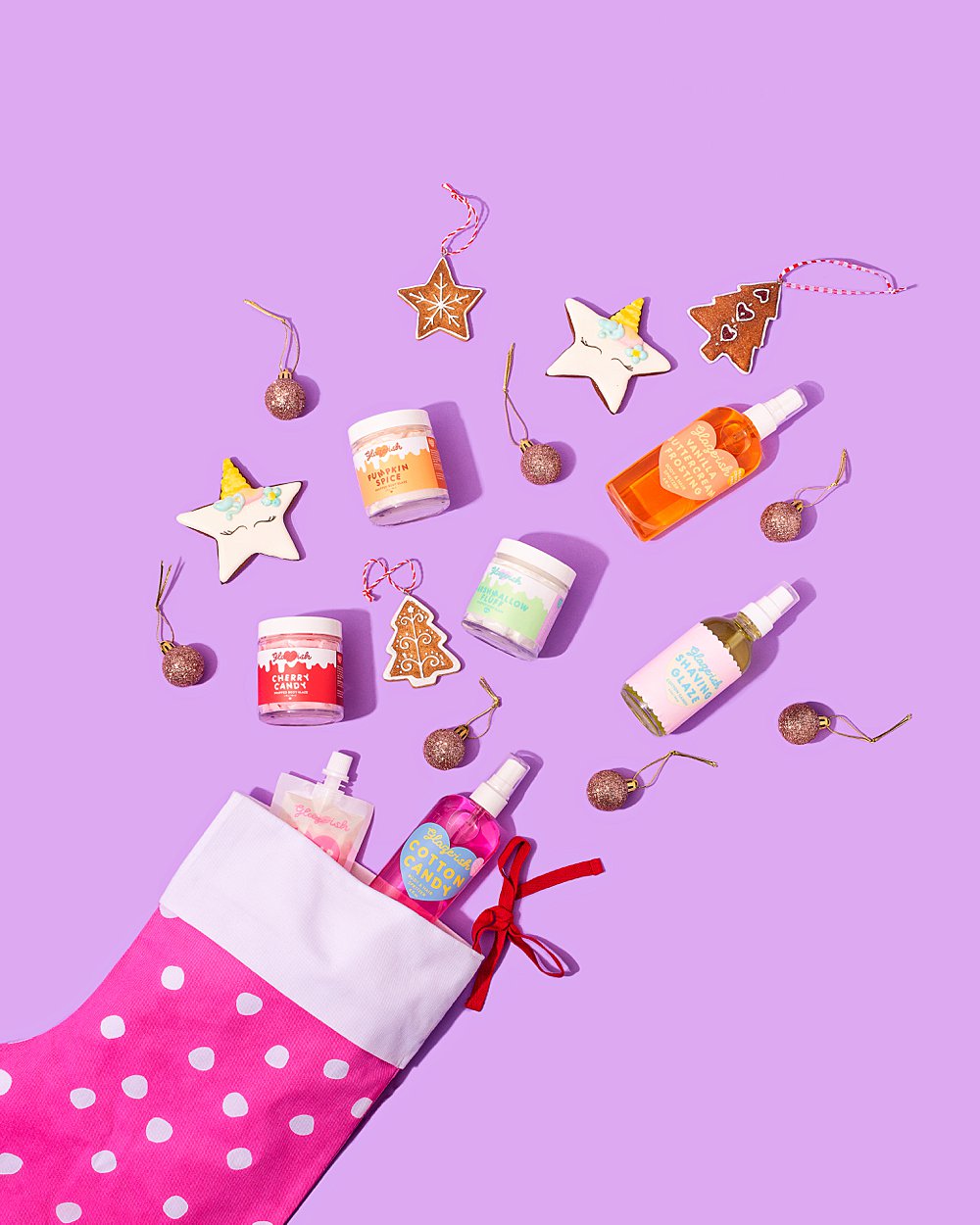The image features a lilac, square background with a festive theme. In the bottom left-hand corner rests a pink and white Christmas stocking, adorned with white polka dots and a white cuff, laying on its side. Emerging from the top of the stocking are multiple beauty products, including bottles and jars with labels like "Cotton Candy," "Pumpkin Spice," "Cherry Candy," "Vanilla Buttercream Frosting," "Shaving Glaze," and "Marshmallow Fluff." Scattered across the surface are decorative ornaments: small gold balls and brown Christmas trees on wires, two gold stars, one bronze star, and what appears to be a snowflake ornament with a brown background. The entire setup on the purple background suggests a holiday-themed marketing display for personal hygiene and beauty products, likely featuring holiday-inspired scents and names.